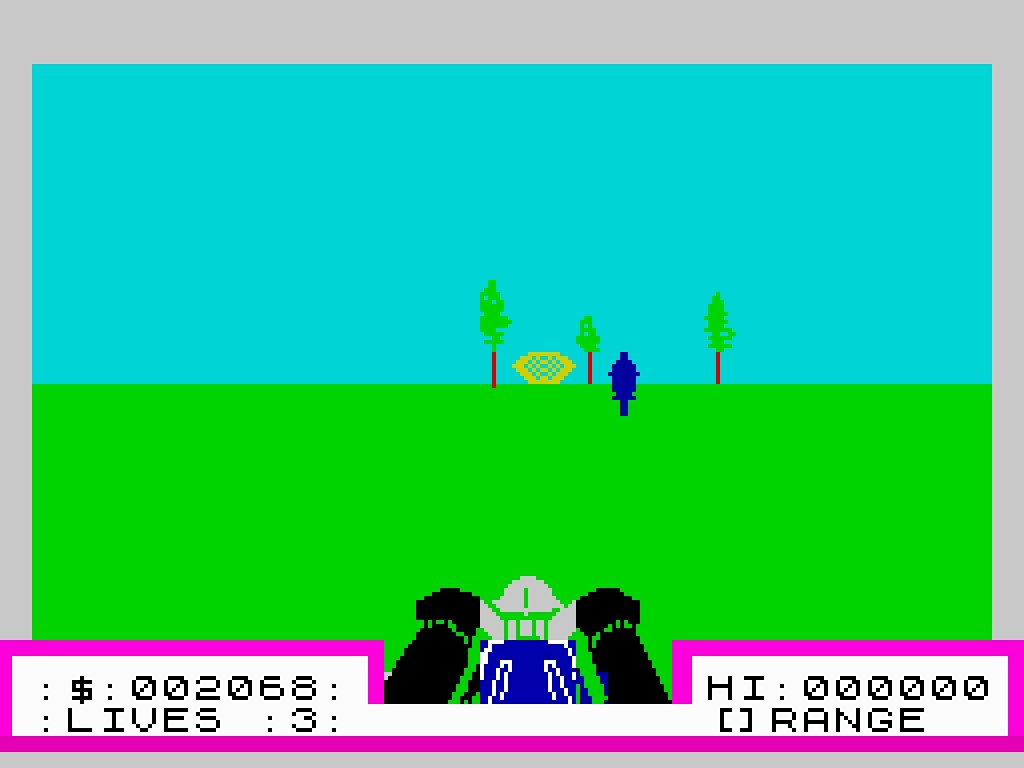This image showcases an antique video game screen, characterized by its retro, pixelated graphics. At the bottom of the screen, the score is vividly displayed in a bright pinkish-purple hue, outlined for clarity. The black print indicates the player's current money and remaining lives. Dominating the center, two black limbs extend from either side, simulating the arms of a soldier clad in blue attire and a gray helmet. The background is a striking neon green that spans the width of the screen, transitioning to a serene blue, possibly symbolizing the sky. Along the lower portion of the screen, three small pixelated trees are arranged from left to right. Between the first and second trees stands a yellow goalkeeper, adding an element of challenge to the scene.